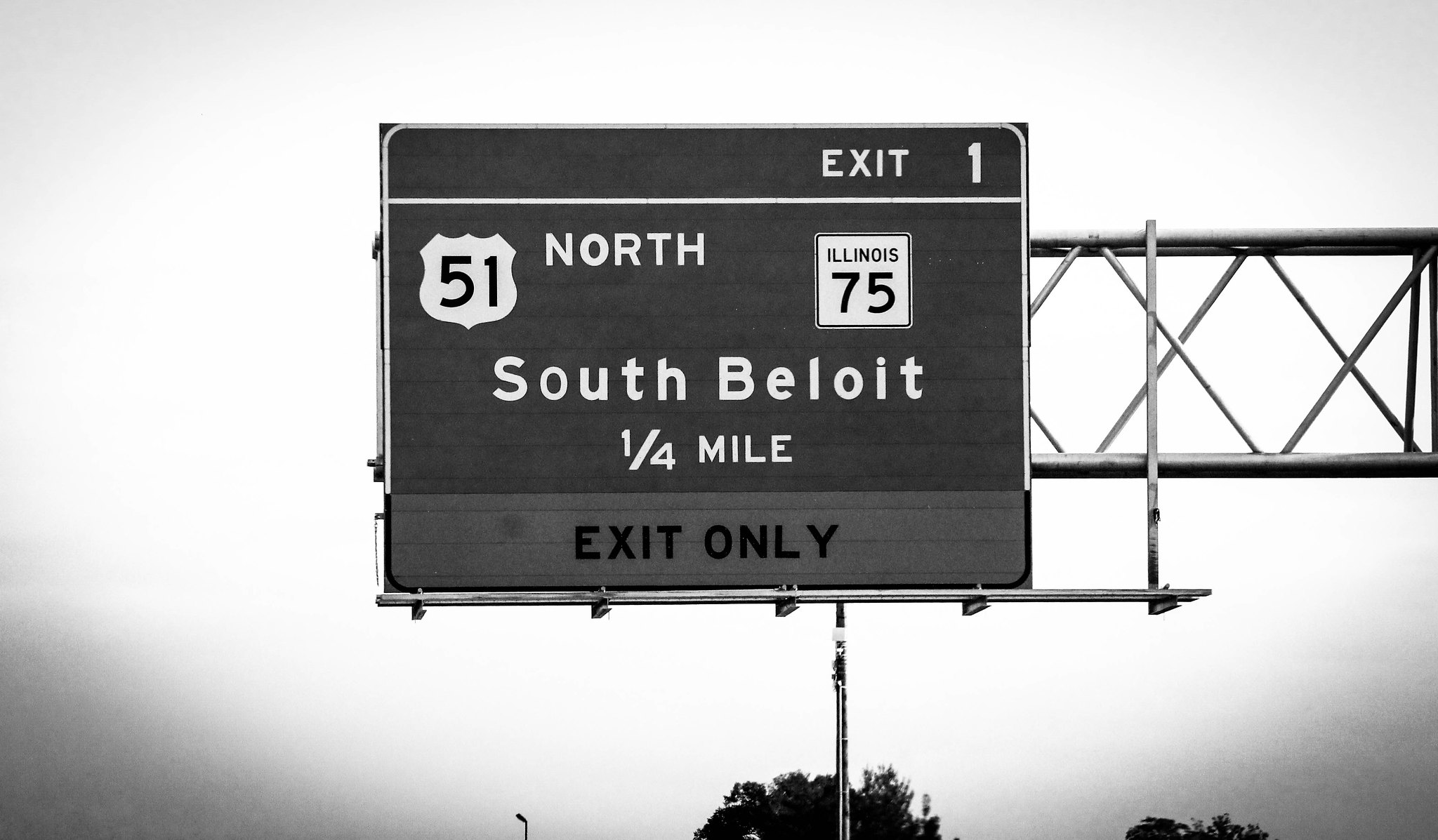The image displays a prominent highway exit sign suspended in the air by metal bars extending from the right side of the frame. The photograph is in black and white, giving a gloomy vibe with a gray, overcast sky. The sign, a large square, includes various directional information: "Exit 1" at the top, "North 51" on the left, "Illinois 75" on the right, and "South Beloit 1/4 Mile" followed by "Exit Only" at the bottom. Despite the illumination coming from the sun, it only faintly brightens the corners, which are heavily vignetted. Below the sign, the tops of trees are barely visible against the dark background, making it hard to distinguish their foliage.